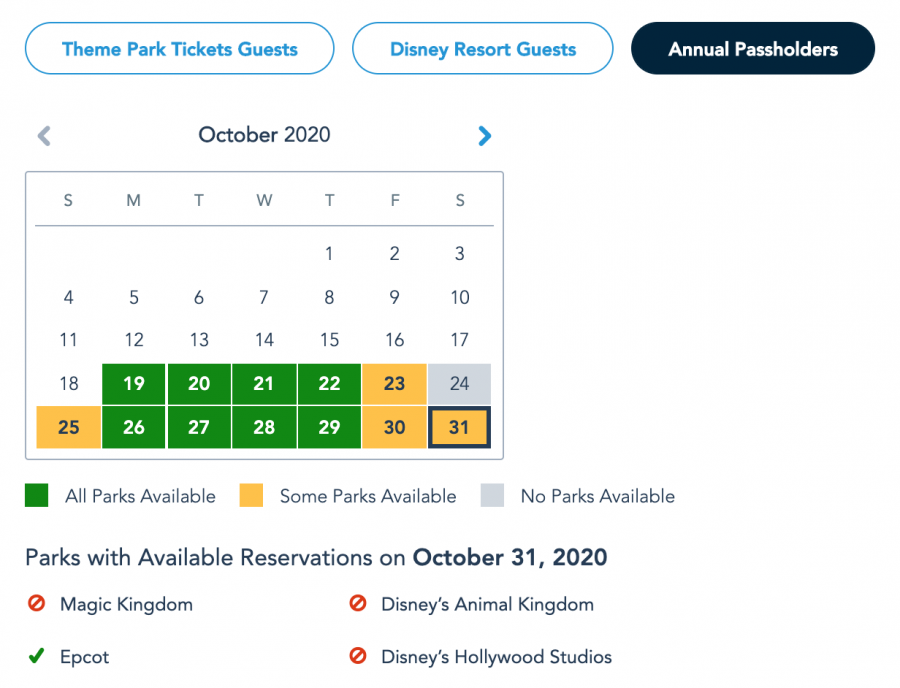This image is a screenshot of a reservation calendar from a website for booking theme park passes and tickets. At the top of the image, there are three oval-shaped icons with blue text. The first icon reads "Theme Park Ticket Guests," the second says "Disney Resort Guests," and the third, which is highlighted in darker blue to indicate it is selected, reads "Annual Pass Holders." 

Directly below these icons is an image of a calendar for October 2020. Navigation arrows are displayed on either side, with a grey arrow pointing left and a blue arrow pointing right. The calendar displays dates with several of them highlighted in different colors: 

- Green (indicating "all parks are available") on the 19th, 20th, 21st, 22nd, 26th, 27th, 28th, and 29th. 
- Orange (indicating "some parks are available") on the 23rd, 25th, 30th, and 31st. 
- Grey (indicating "no parks are available") on the 24th.

A key below the calendar explains the meaning of the colors: green boxes mean all parks are available, orange boxes mean some parks are available, and grey boxes mean no parks are available.

At the bottom of the image, there is a list under the heading, "Parks with available reservations on October 31st, 2020." It shows a no-entry symbol (indicating no available reservations) next to Magic Kingdom, Disney's Animal Kingdom, and Disney Hollywood Studios. A green check mark next to Epcot indicates that reservations are available for this park on October 31st.